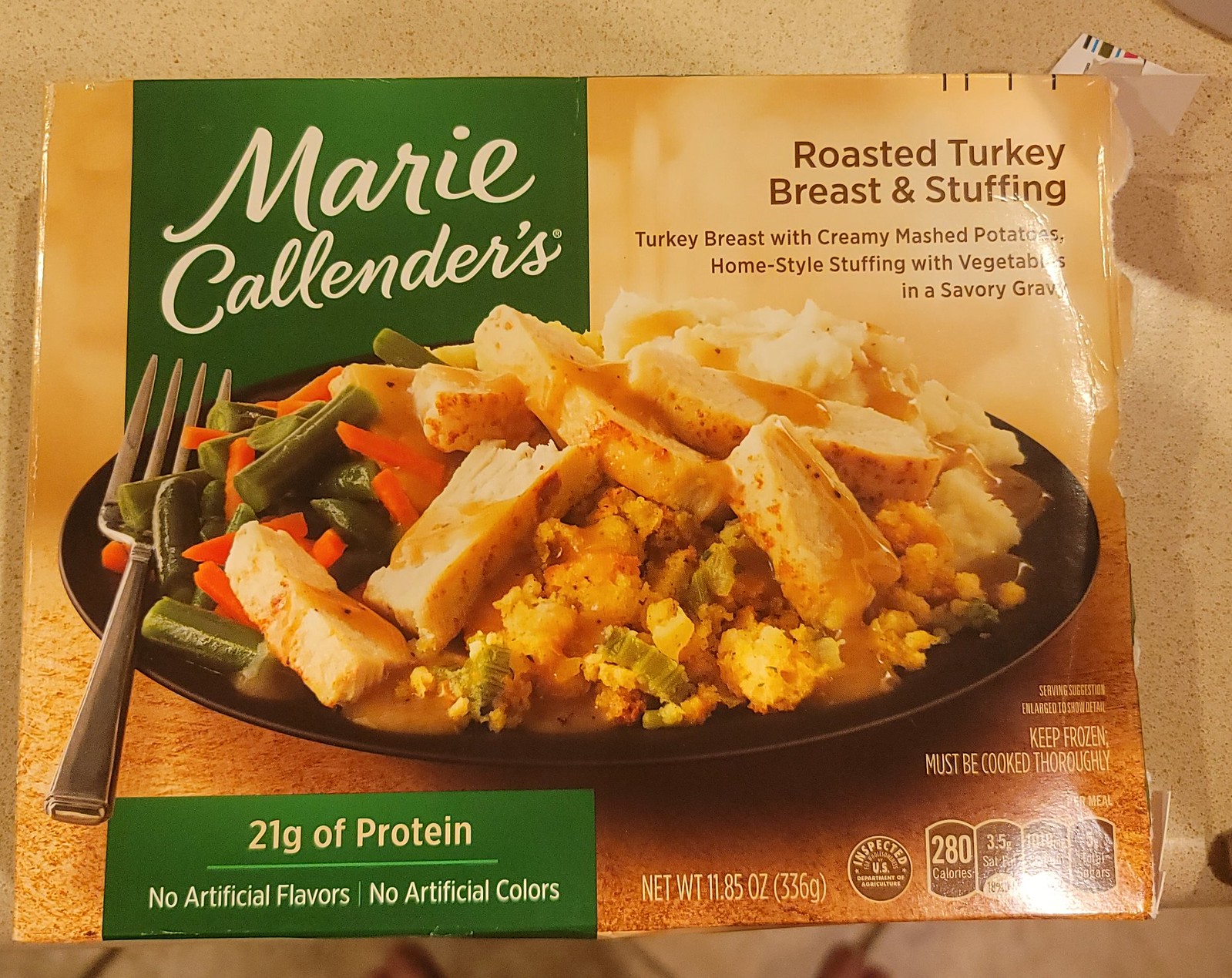This image features a Marie Callender's Roasted Turkey Breast and Stuffing meal, showcased against a tan background. The packaging displays a delectable meal arranged on a black plate, with a fork placed to the side. The plate contains tender chunks of roasted turkey breast, some broken to reveal their texture, accompanied by mashed potatoes drizzled with rich gravy. Next to the turkey and potatoes, there is a portion of flavorful stuffing, also accentuated with a touch of gravy. The plate is garnished with vibrant green beans and bright orange carrots, adding a splash of color to the meal. The packaging highlights key nutritional information, stating that the meal provides 21 grams of protein and contains no artificial flavors or colors. Important handling instructions are also noted, indicating the meal must be cooked thoroughly and kept frozen. The net weight of the meal is clearly indicated at the top, though some of the writing is not clearly visible.